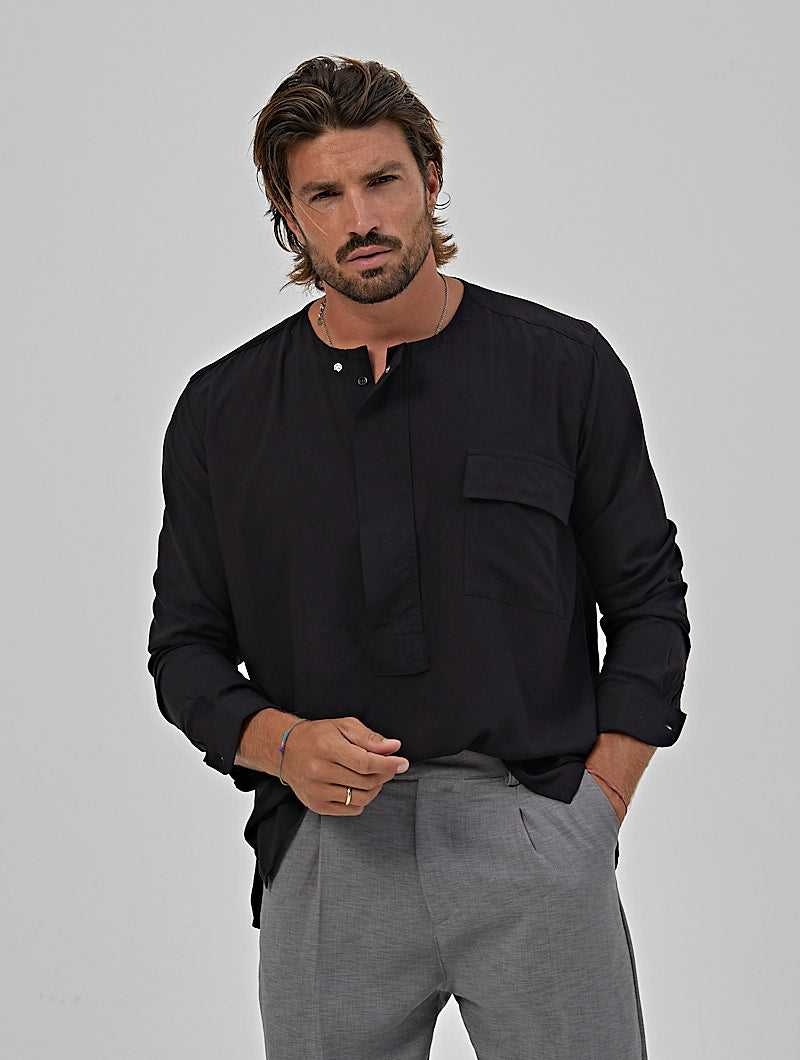The photograph features a male model standing in front of a neutral background. He exudes a pensive demeanor as he looks directly at the camera. His long, lightly highlighted brown hair is slicked back, reaching the nape of his neck, complementing his neatly trimmed beard and mustache. He is dressed in a black, long-sleeved, linen-like blouse with an open round collar and a noticeable pocket on the left side. His attire is completed with light gray, pleated slacks. The model's right hand rests in his pocket, while his left hand is positioned in front of his waist, showcasing a gold wedding band on his ring finger and a colorful bracelet on his wrist. He also wears a subtle gold chain around his neck and has a slightly tanned complexion.